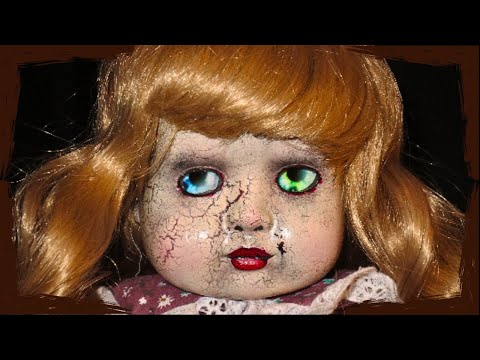This image features an antique, creepy porcelain doll with a heavily detailed and unsettling visage. The doll's once shiny, beige-colored face is now tarnished, displaying numerous cracks which reveal a reddish base underneath the deteriorating paint. Its facial features include a small nose, stark red painted lips, and a pair of mismatched eyes that draw immediate attention due to their eerie nature. The left eye is a jeweled blue, while the right eye is green; both eyes appear blurry and cloudy, accentuating the doll’s sinister appearance. The eyes are surrounded by black shaded eyebrows and a hint of red around the outlines. The doll's hair is a reddish-copper tone, with bangs that hang over its forehead and the rest styled into almost ponytail-like sections. This figure is dressed in a wine-colored fabric dress, adorned with white cloth flares and patterned designs. The background is very dark, almost black, bordered faintly by brown, which adds to the ominous atmosphere of the image. Black bars on the top and bottom of the image frame the zoomed-in focus on the doll’s face, making the overall composition even more unsettling.